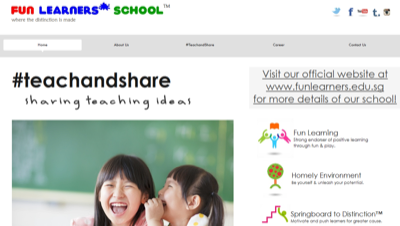A screenshot of the Fun Learners School website displays a clean, predominantly white background. In the upper left corner, vibrant capital bubble letters spell out "Fun Learners School" with "Fun" in red, "Learners" in blue, and "School" in green. Beneath the name, the tagline, "Where distinction is made," is written in black. The top-right corner features old logos for Twitter, Facebook, YouTube, an unidentified "T" logo, and Instagram.

Below this, a gray menu bar presents five options, with the leftmost option highlighted in a white square labeled "Home." The following option is "About Us." The third and fourth options are unreadable, while the last option reads "Contact Us."

The main image on the page captures a joyful moment between two Asian girls, one whispering into the other's ear, against a blurred green chalkboard backdrop. Positioned above the image is the hashtag "#TeachAndShare" in black, followed by the phrase "Sharing Teaching Ideas."